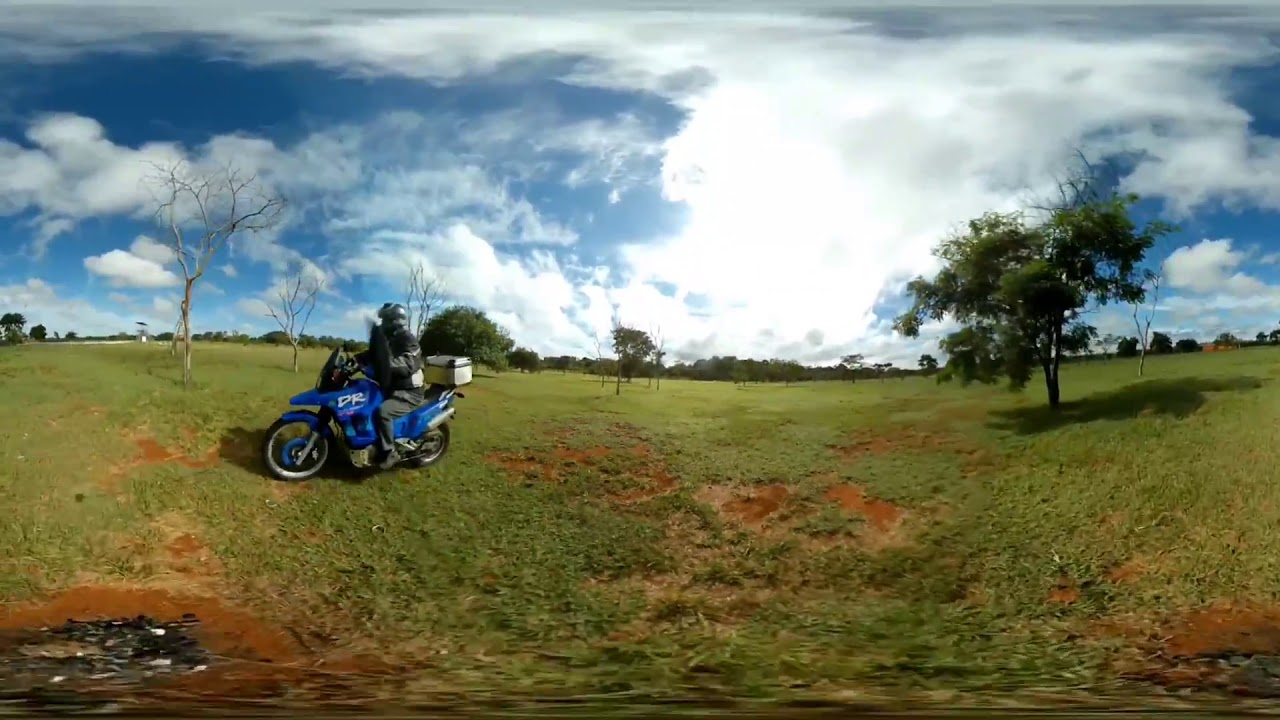In this photograph taken outdoors, a vast grassy field stretches out, peppered with patches of rusty red clay-like dirt. The setting captures an early spring atmosphere, evident from the mix of bare branches and leafy trees that line the background. Central to the image, positioned slightly to the left, is a person on a blue motorcycle, facing left. The motorcycle, side-viewed, features the letters "DR" in white and has a light-colored box attached at the back. The rider is geared up in a black leather-like jacket, gray pants, and a silver helmet. The sky above is a blend of blue and gray, heavily strewn with clouds, suggesting a mostly overcast day. Some scattered stones or shiny objects can be seen in the foreground to the left, adding to the tactile detail of the scene. There is no text visible anywhere else in the image.